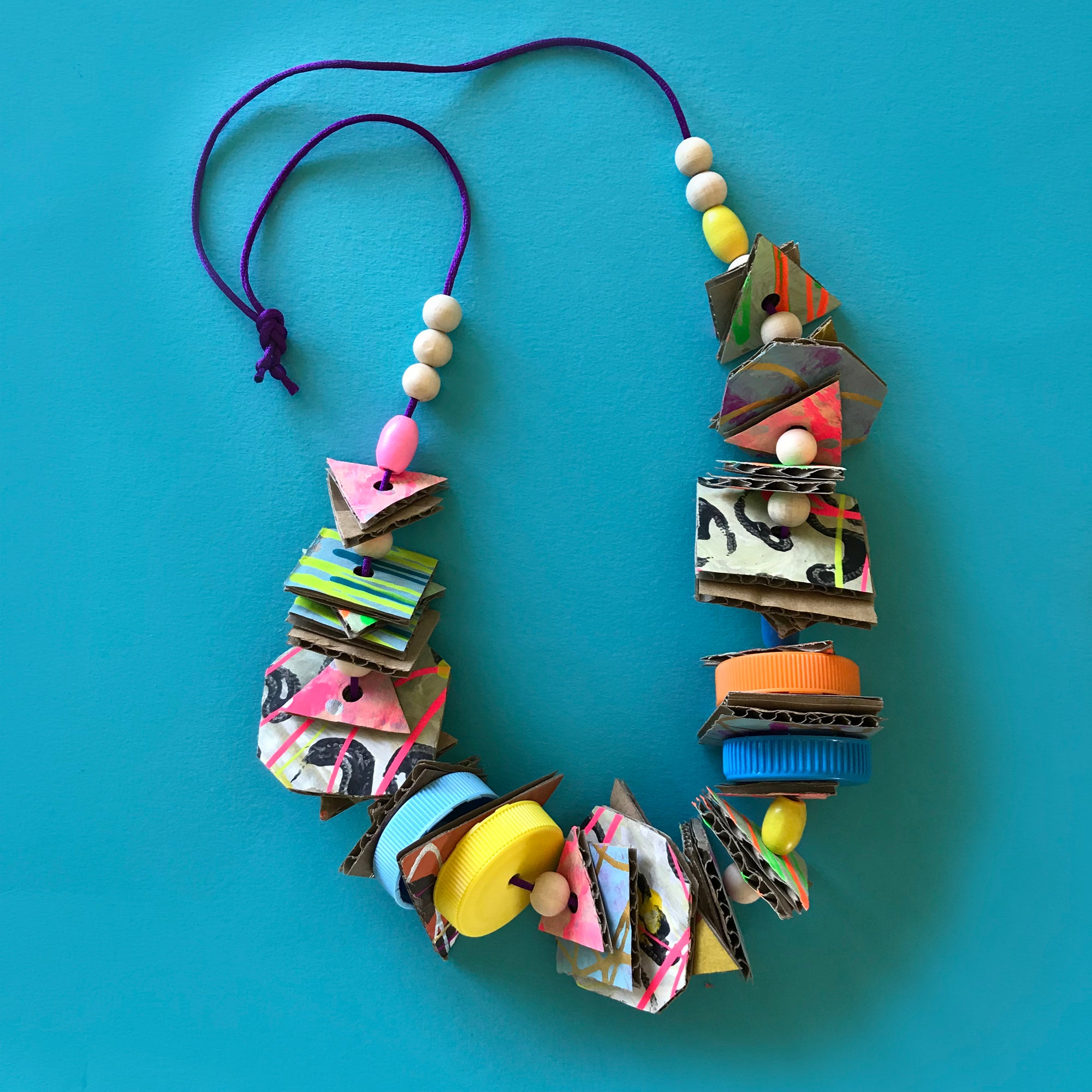The image showcases a vibrant and colorful handmade necklace, set against a teal background. The necklace features a striking purple cord tied at the top, adorned with various recycled materials. It includes multiple sections of painted cardboard cutouts, fashioned into triangles and squares with hues of pink, blue, green, yellow, and black. These cutouts are interspersed with an array of beads and upcycled bottle caps. The beads are a mix of wooden and plastic, with three beads on each side—a combination of wooden and pink plastic beads on the left, and wooden and yellow plastic beads on the right. The cardboard pieces are punctuated by brightly painted bottle caps in shades of turquoise, yellow, orange, and blue. Centrally located on the necklace is an unpainted wooden bead accompanied by a small yellow plastic bead, adding to the intricate detail of this sustainable, artistic jewelry piece.